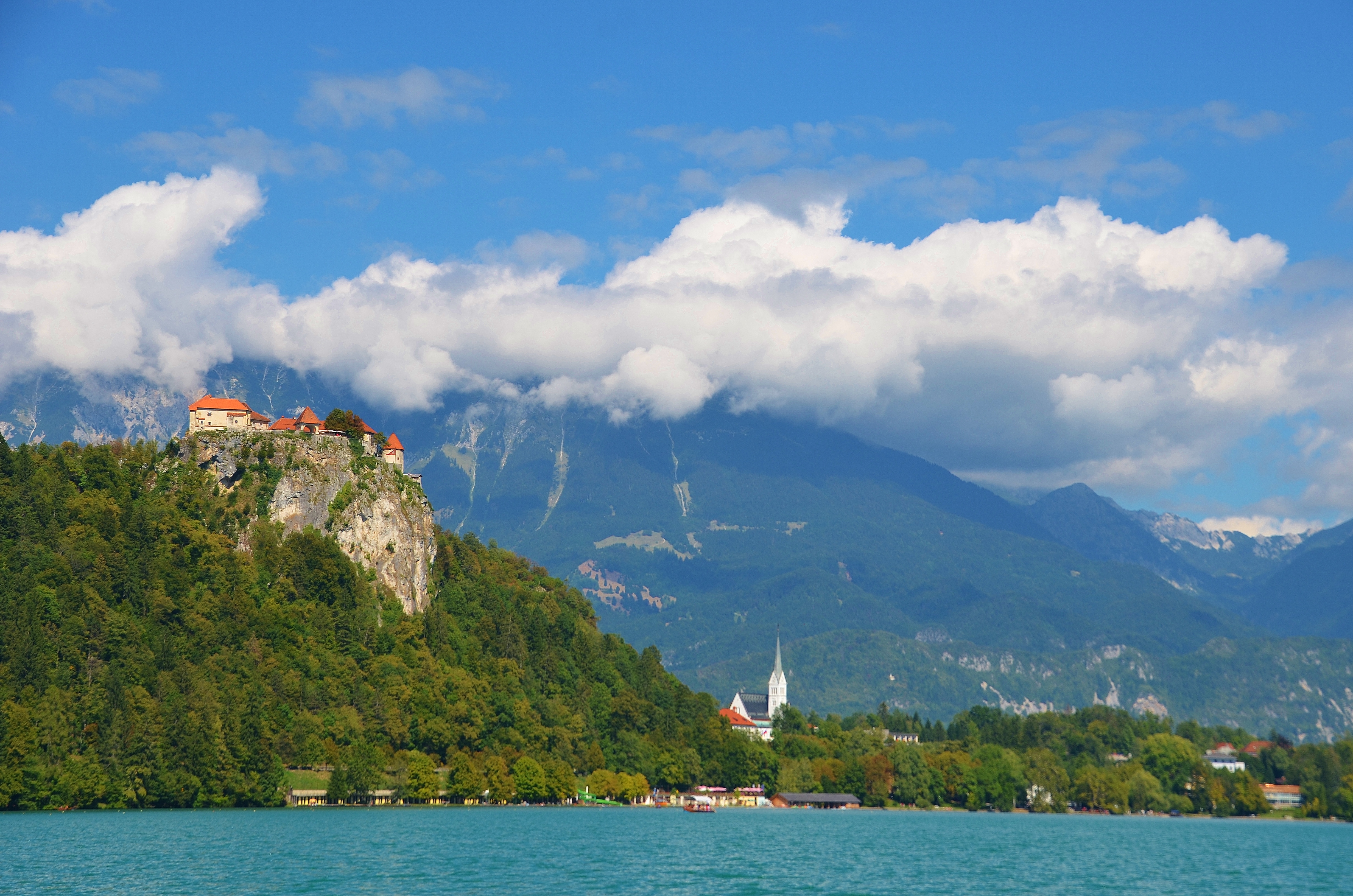This landscape-oriented photograph captures the serene beauty of Lake Bled in Slovenia. Taken from a vantage point on the water, the image unfolds a mesmerizing scene. The lower portion, approximately one-eighth of the frame, showcases the calm yet slightly rippled surface of the lake, shimmering in a tranquil aqua blue.

To the right, the majestic mountains rise dramatically, covered in lush greenery that hints at the rich vegetation of the region. These towering peaks frame the image, their rugged forms contrasting beautifully with the gentle waves below. The top half of the photograph is dominated by an expansive sky, a brilliant blue canvas adorned with a scattering of white, fluffy clouds that seem to float just above the mountaintops.

Drawing the eye to the left-hand side, the lush, green mountain slopes further define the scene. Nestled at the end of this verdant expanse sits a picturesque castle, adding a touch of historical charm and intrigue to the landscape. This architectural gem seems to stand sentinel over the serene waters, completing a breathtaking scene of natural and man-made beauty.